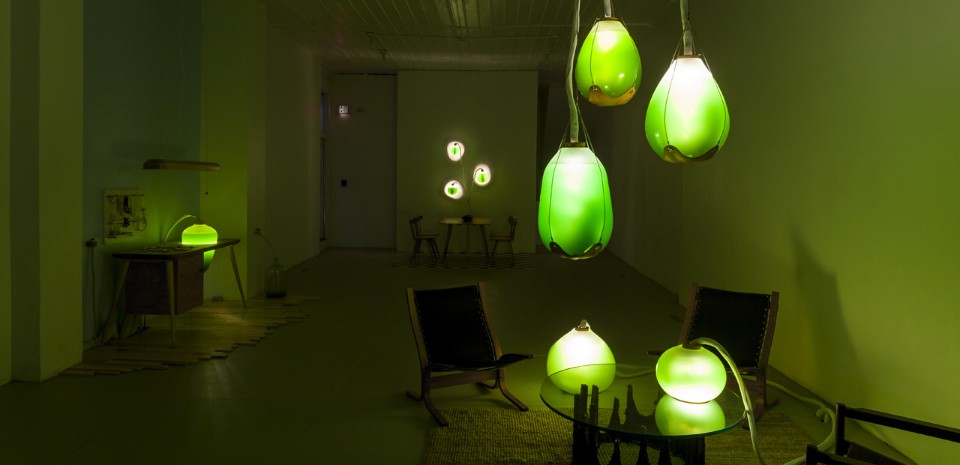The image depicts a dimly-lit, sparsely furnished room that appears to be either a large living room or a minimalist apartment. The room is dominated by green lighting, casting a pea-greenish hue on the walls and furniture. The central focus is on the multiple green chandelier lights hanging from the white-tiled ceiling, and individual green lamps scattered throughout the space. 

In the foreground, on the right, a glass table holds an illuminated green orb, and nearby, several low hammock-style black chairs rest on a Hessian rug. Another glowing green orb sits on the floor beside them. In the middle ground to the left, a brown animal-skin style rug supports a wooden desk, which also features a green lamp. Tools hang on a small white pin-style storage solution mounted on the wall above this desk.

Towards the back of the room, a wooden table with three green bulbous lamps is flanked by two wooden chairs, one on each side. There is a closed door on the far left and an open doorway on the far right, adding to the room's spacious yet sparse feel. The array of green lights is the prominent feature in this almost empty apartment, accenting the minimalistic furniture setup and enhancing the room's unique aesthetic.